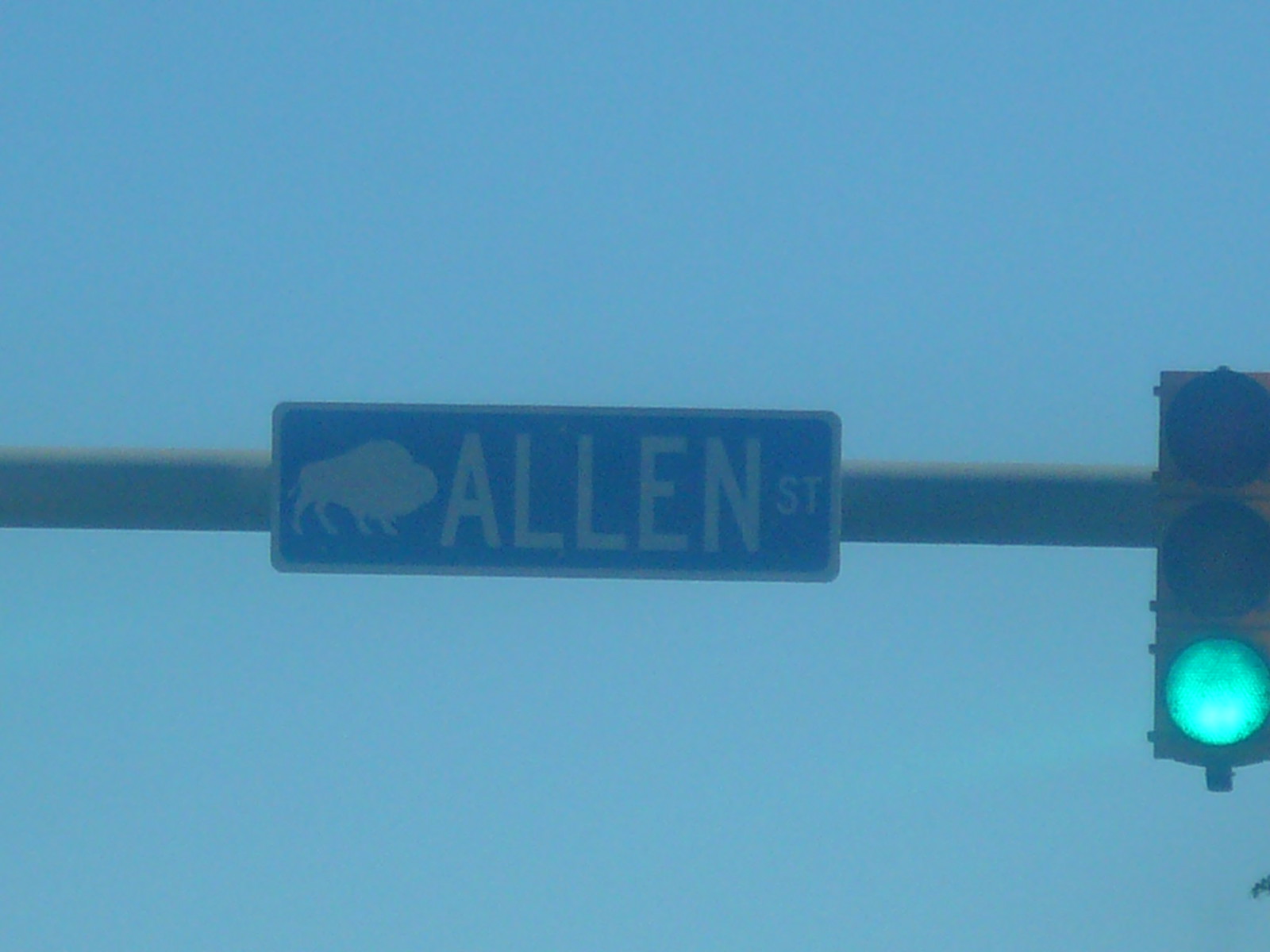A blurry, enlarged image depicts a silver street light post with a green traffic light attached. Adjacent to the street light is a blue road sign with the white, albeit darkened, text 'Allen St', with 'Allen' being significantly larger than 'St.' An animal figure is seen near the 'Allen' text, adding an intriguing element to the scene. The backdrop features a clear, blue sky, suggesting a lovely day despite the photo's lack of sharpness.